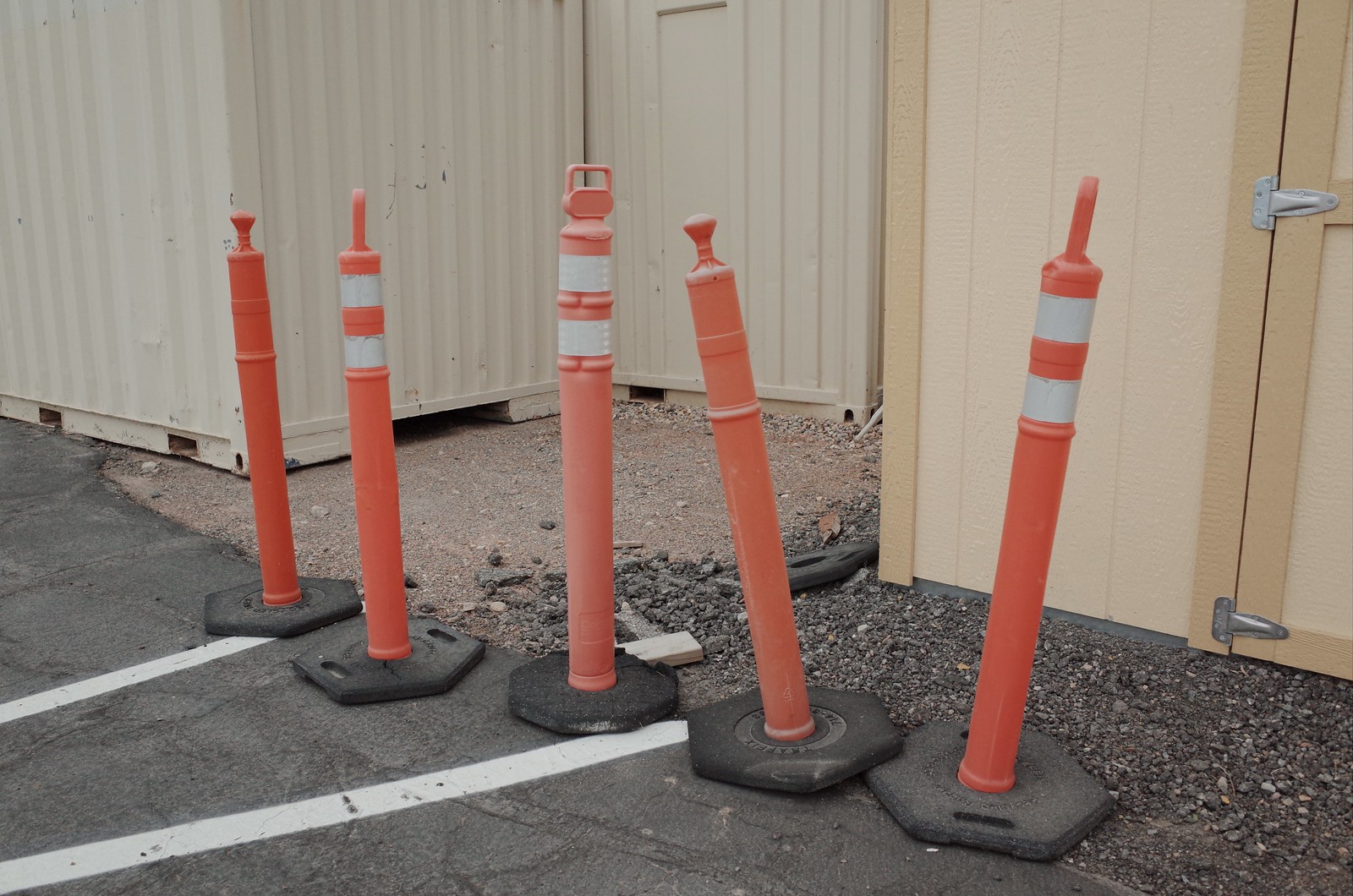This image captures a gravel and dirt parking lot situated in front of cream-colored temporary storage units, likely shipping containers, one of which has a visible door on its right side. The foreground reveals an asphalt area with two white painted lines, suggesting designated parking spaces. Central to the image are five bollards with black hexagonal bases and orange vertical posts, three of which have two white reflective stripes near their tops while the remaining two lack the reflective material. The scene appears to be set on a cloudy day as indicated by the absence of shadows. Additionally, the right side of the image includes a wooden shed-like structure with a door, enhancing the impression of a construction site or a makeshift storage area.